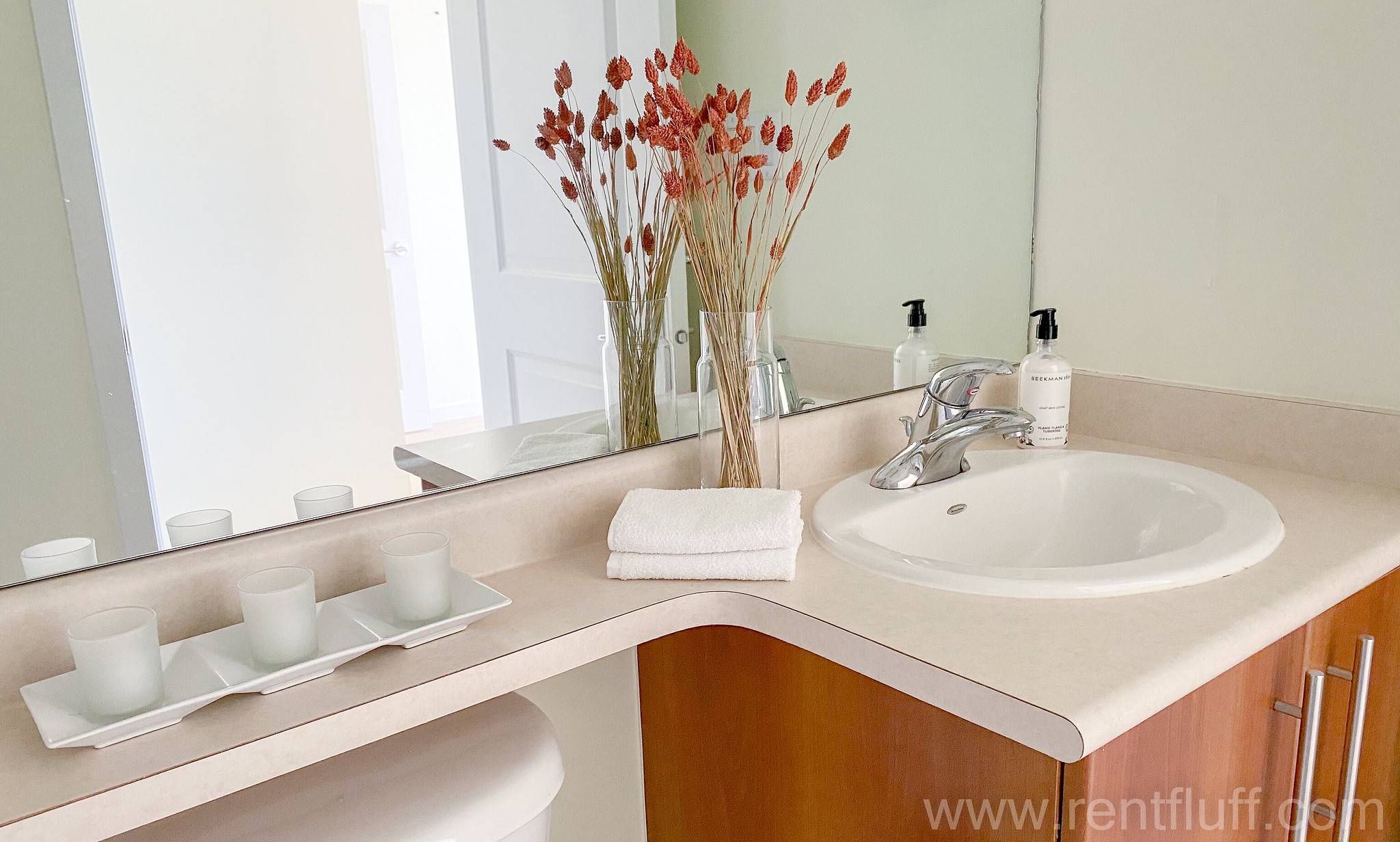The image showcases a neatly organized and aesthetically pleasing bathroom. On the right side, a white wall frames the space, creating a clean and fresh backdrop. The countertop, positioned in the corner to the right, is off-white and supports several functional and decorative items. Set into the countertop is a pristine white sink, accentuated by a sleek chrome faucet with a simple left-right mechanism for temperature control.

To the right of the sink stands a pump bottle, presumably filled with hand soap. On the left side, a clear glass vase contains dried foliage with brown stalks and rust-colored heads, adding a touch of naturalistic charm. Nearby, two white hand towels are neatly folded.

Below the countertop, a wooden cabinet with silver handles provides storage space through its two-door design. The countertop extends slightly along the adjacent wall, hosting three white, interconnected plates that serve as frosted candle holders. Beneath this extended counter space sits the top of a white toilet, completing the tidy and harmonious bathroom setup.